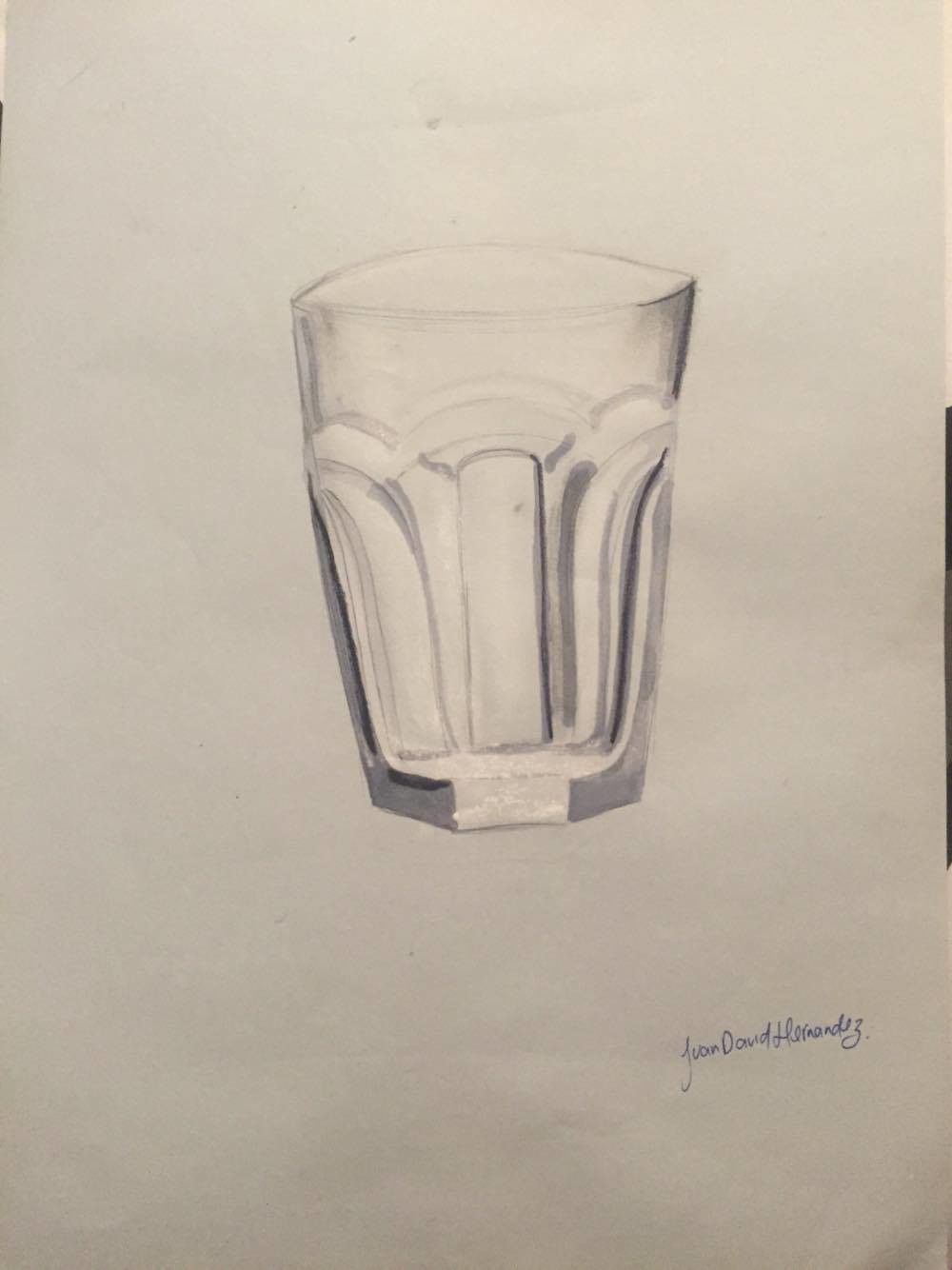A highly realistic pencil sketch of an empty bar glass is meticulously drawn on a pristine white sheet of paper. The bar glass, traditionally used for beverages like water, soda, tea, or possibly beer, features intricate detailing. It has indented designs around the middle, contrasted by a smooth upper section, and rests on a clear glass base, showcasing the artist's remarkable shading techniques that bring lifelike depth and dimension to the piece. The entire artwork is rendered in black and white, emphasizing the precise and careful use of pencil. The artist has signed their work in cursive at the bottom right corner, adding a personal touch to this exquisite sketch.